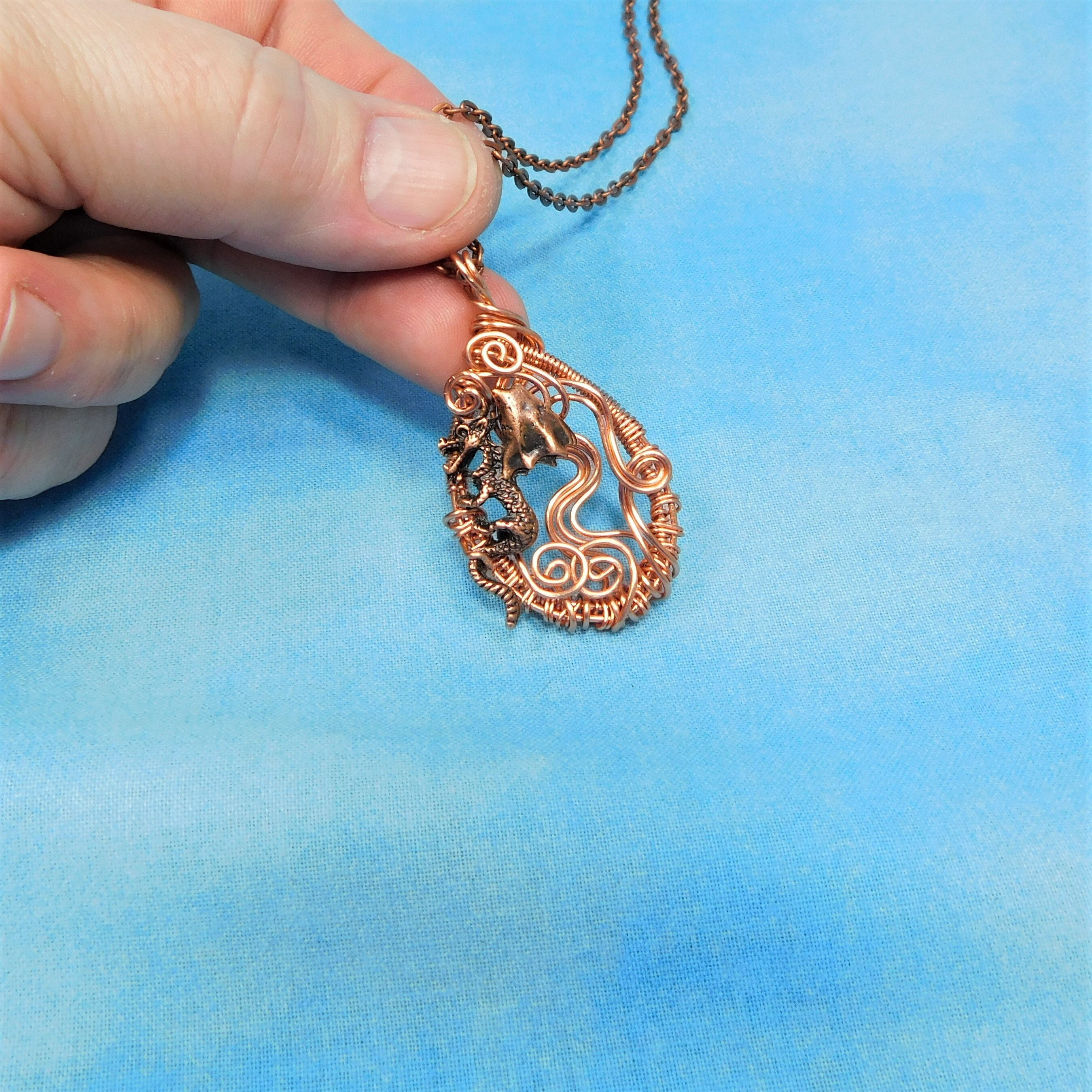In this staged, square, full-color indoor photograph, a Caucasian left hand with short fingernails is prominently visible in the upper left corner, pinching a necklace at the pendant. The background appears as a light blue fabric with blends of white, reminiscent of a sky. The necklace features a very thin gold chain that curves gently before disappearing out of the frame. The chain holds a teardrop-shaped pendant with a gold wire border wound around its edges. The pendant itself has ornate, intricate swirls forming abstract patterns resembling a dragon or perhaps a squid, with tentacle-like curls extending within the design. The overall impression is one of delicate craftsmanship, with the hand displaying the intricate beauty of the necklace against the soft, blended backdrop.